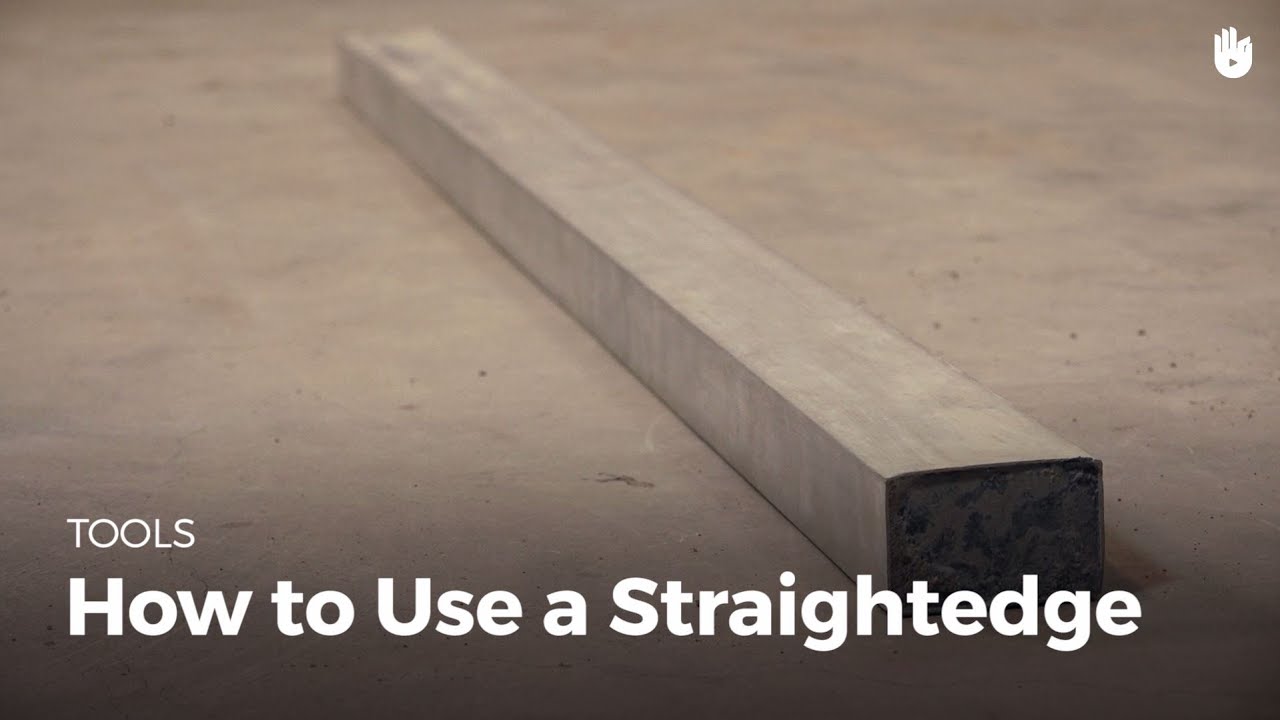The image depicts a slightly aged and speckled concrete or cement surface, which could either be a ground or a flat table. Diagonally spanning from the lower right to the upper left corner is a large wooden beam, possibly a 2x4, cut evenly at both ends and colored gray. In the lower left corner, the image features bold, white capital letters stating "TOOLS," with the subtitle "How to Use a Straight Edge" positioned just below it in white text. The upper right corner of the image contains an icon resembling a hand, with the thumb and pointer finger touching, accompanied by an arrow pointing to the right. This appears to be a thumbnail for an instructional video or tutorial on using a straight edge.